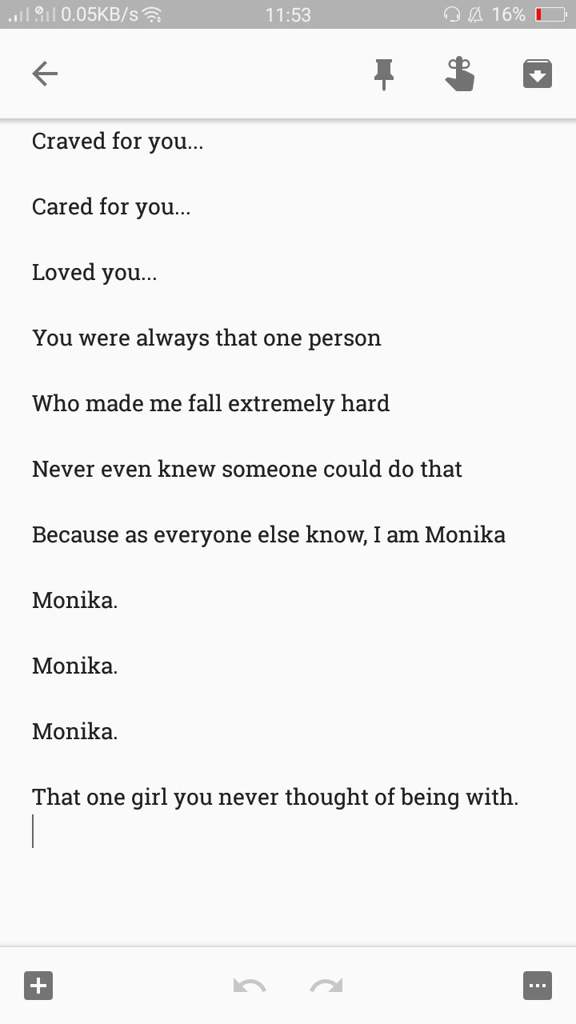A poignant screenshot captured on a mobile phone displaying a heartfelt note in a note-taking app. The note reads, "Craved for you, cared for you, loved you. You were always that one person who made me fall extremely hard. Never even knew someone could do that. Because as everyone else knows, I am Monica, Monica, Monica, Monica. That one girl you never thought of being with." The screen's status bar shows the battery level at 16%, indicating low power, and the phone is on silent mode with headphones connected. The time displayed is 11:53 AM. Various icons in the upper left corner indicate the phone's signal strength. At the bottom of the screen, there are additional app controls; a plus sign on the lower left for adding new content, three vertical dots on the lower right likely for more options, and undo and redo buttons in the center for editing notes.